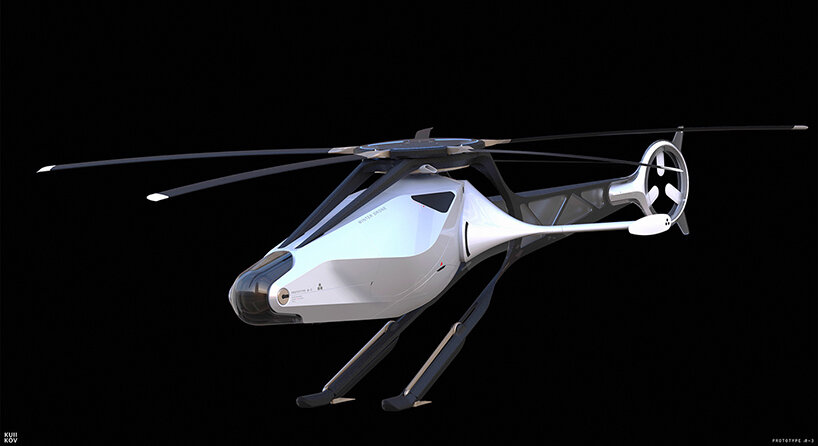This image showcases a detailed artist’s concept of a futuristic design for a helicopter, set against a plain, solid black background. The rectangular image, approximately 5 inches wide by 3 inches high, features a computer-generated or AI-rendered helicopter. The helicopter's design is notably sleek and minimalist, characterized by a black-and-white color scheme with hints of blue on top.

The main rotor at the top consists of four blades, which are gray with white tips. The helicopter's body is predominantly white with a dark gray or black nose. Notably, the design eschews conventional pilot visibility, as it lacks visible windows. A small, thin wing extends from the right-hand side of the fuselage, ending in a rounded tip. The black tail extends backward, segmented with what appear to be cut-out sections to keep the design lightweight, ending in a circular component with fins inside.

Supporting the body are two slender legs, likely designed for lightweight mobility, with small foot areas. Additionally, both the legs and the helicopter's propellers are black, contrasting with the predominantly white body. The image includes small, indistinct white text in both the lower left and lower right corners, possibly indicating labels or technical details such as “prototype” or creator initials, which could be interpreted as “KUM KOV” or something similar. This high-tech concept art evokes the aesthetics of a sci-fi movie or video game, emphasizing a streamlined and futuristic appearance.